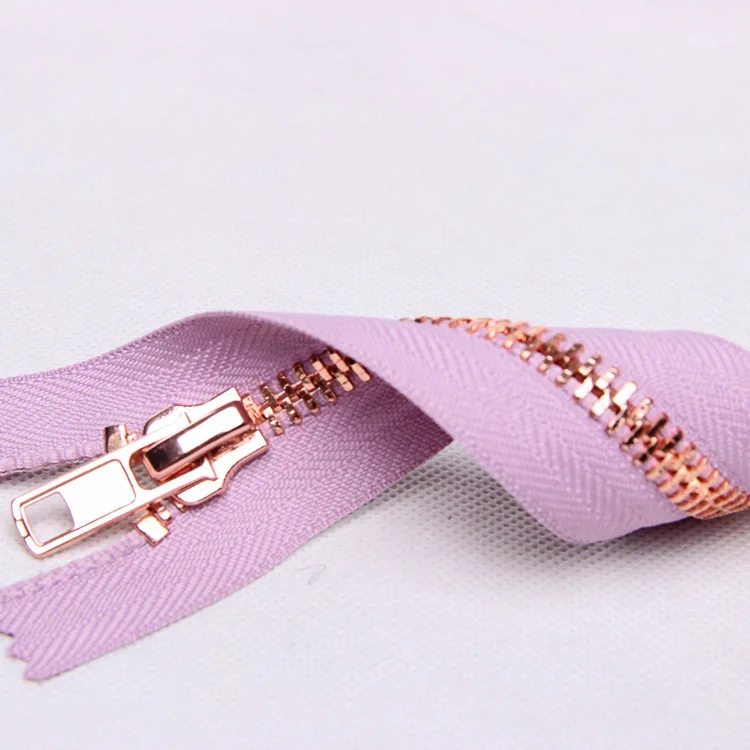The image features a striking, shiny gold-colored zipper that appears new and highly polished, running horizontally across the center of the frame. The zipper is securely attached to a narrow strip of fabric that has a pinkish-purple hue, with the specific shade varying slightly between pink and purple tones. This fabric displays a subtle textured pattern with diagonal lines, enhancing its visual appeal. The fabric twists and curls slightly, showcasing both the front and the back of the zipper, adding a dynamic element to the composition. The background is a light to medium gray square, possibly textured or shadowed, providing a neutral yet sophisticated backdrop that highlights the zipper and its attached fabric strip. No text is present in the image, allowing the focus to remain solely on the elegantly displayed zipper and fabric.